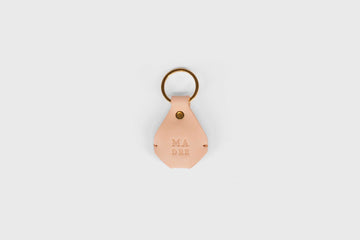The image displays a keychain with a brown-colored loop supporting a light pink leather pocket. The pocket is inscribed with the word "MADRE" in embossed letters, adding texture to the design. The background of the image is a soft light gray, enhancing the delicate pastel tones of the pink pocket. The pocket somewhat resembles a dog tag, featuring small dots on either side that add further detail. The keychain is accented with a brass ring, providing a subtle contrast against the lighter colors. Overall, this simple yet elegant keychain stands out against its white and gray backdrop, highlighting the craftsmanship and thoughtful design of the piece.